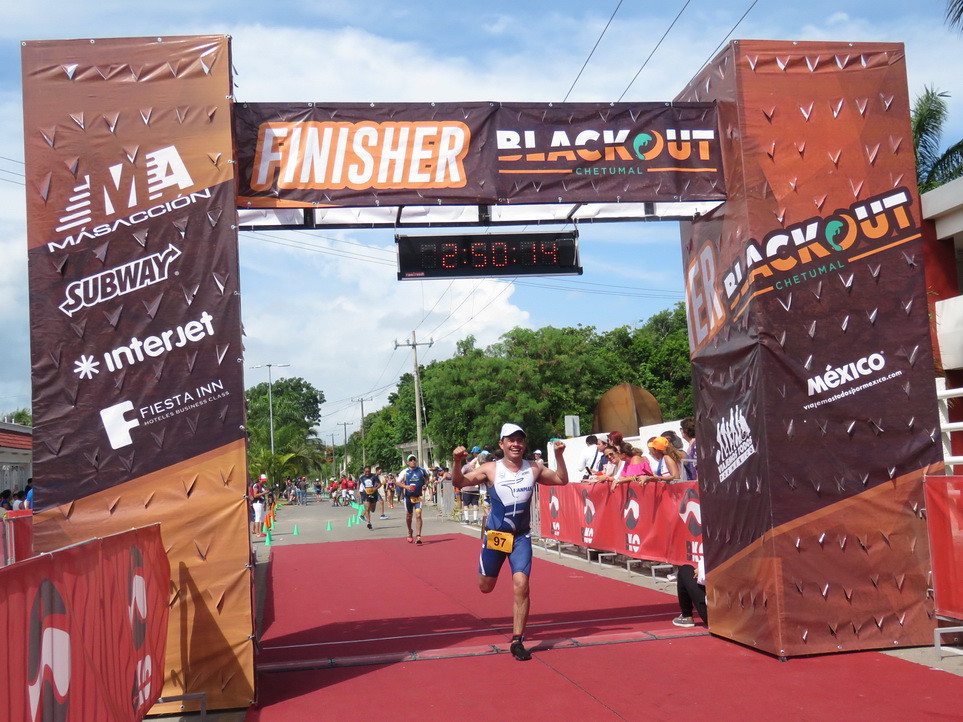In this detailed image from a marathon race event held outdoors in the middle of the day, we see a stone concrete ground with a red carpet running down the center of the track, leading to a finish line archway. The finish line structure consists of two tall, square, dark brown columns supporting a rectangular bar overhead. The bar prominently features the word "Finisher," along with various texts and logos, including "Blackout," "Chetumal," and "Mexico." Several sponsors' banners are visible, such as Interjet, Subway, and Fiesta Inn. A digital timer hanging from the top of the archway displays the time "2:50:14." 

Central to the scene is a triumphant runner crossing the finish line. He is wearing a white hat, a blue and white spandex uniform with a gold square and the number 97 in the center. He has both arms raised in victory, with his right leg trailing off the ground behind him. Behind this leading runner, other racers are visible, along with spectators cheering from the sides. Lush green trees and a clear blue sky with some white clouds form the backdrop, adding to the vibrant atmosphere filled with colors like light blue, gray, white, brown, red, yellow, blue, pink, and orange.